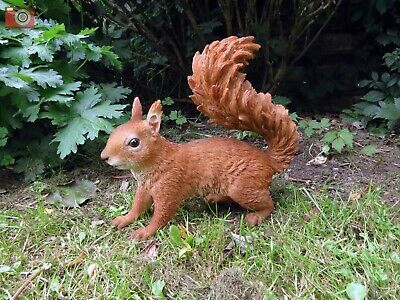The picture features a lifelike statue of a squirrel, intricately detailed to resemble a real one. This small, reddish-brown sculpture is situated on a patch of green grass near the edge of a forest, surrounded by an ombre of leaves that transition from bright green on the left to darker shades on the right, creating a shadowed effect. The statue has a bushy, S-shaped tail, distinctive white markings on its chest and mouth, and black eyes that add to its alert expression, as if it were reacting to a distant sound. The background includes larger leaves and foliage, further enhancing the natural setting of the scene. This highly detailed statue could easily be mistaken for a live squirrel, standing on all fours with perky ears and poised as if ready to move.